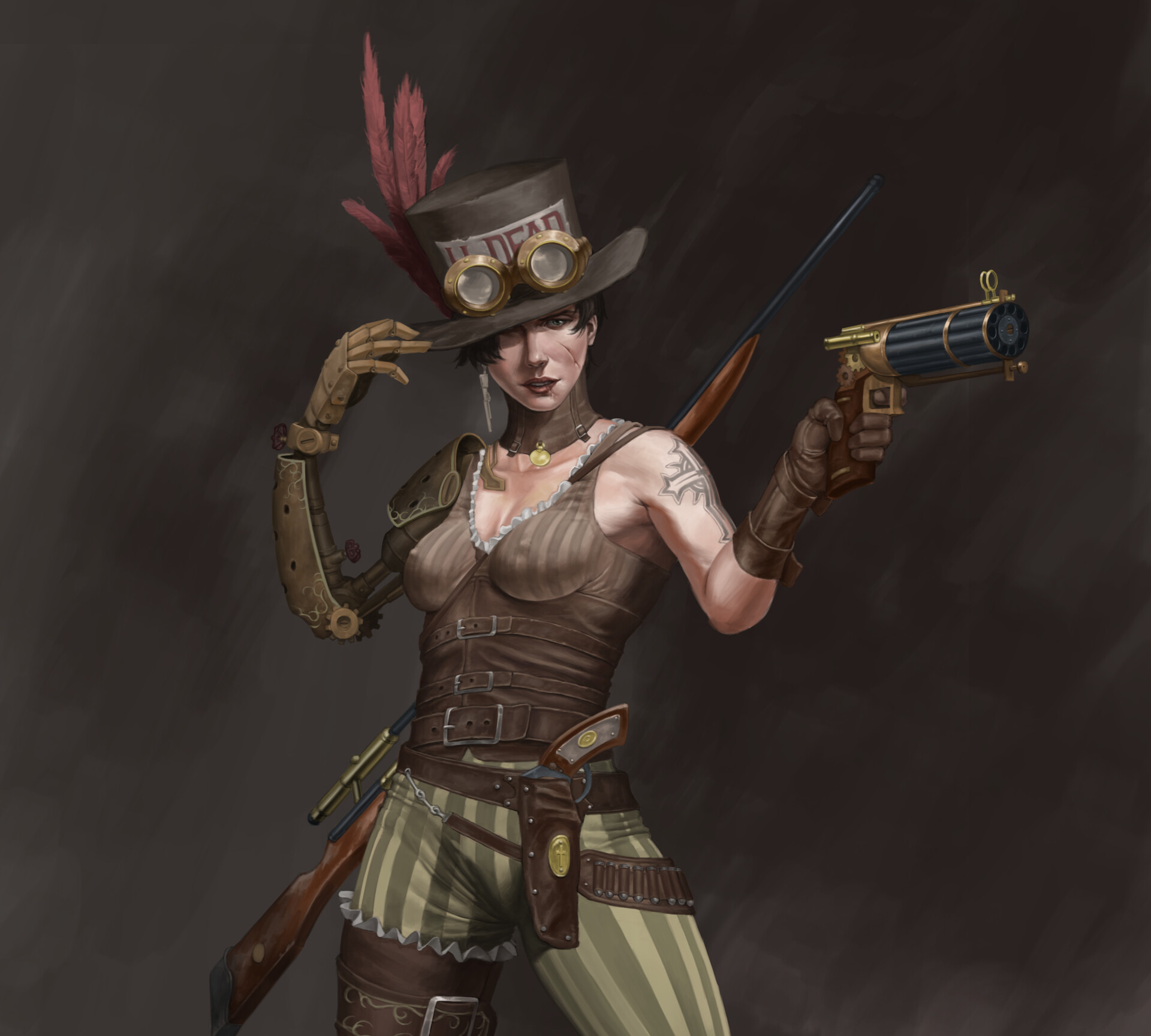The image depicts a steampunk-inspired woman adorned in an intricately detailed outfit dominated by shades of brown and green. She is captured from the knees up, standing against a brown distressed backdrop. Her ensemble features a brown striped corset and green and white striped pants, accessorized with a belt holding various tools. She dons a brown top hat adorned with maroon feathers and goggles, with the word "dead" inscribed on it, and sports a tattoo on her left cheek. Her right arm is robotic, while her left arm, clad in a brown leather glove, holds a small, futuristic-looking pistol. Slung across her back is a larger, old-fashioned gun, and a brown boot is visible on her right foot. The overall aesthetic of the image leans heavily into the steampunk genre, blending elements of historical style with mechanical and futuristic nuances, giving it a digital artwork feel.